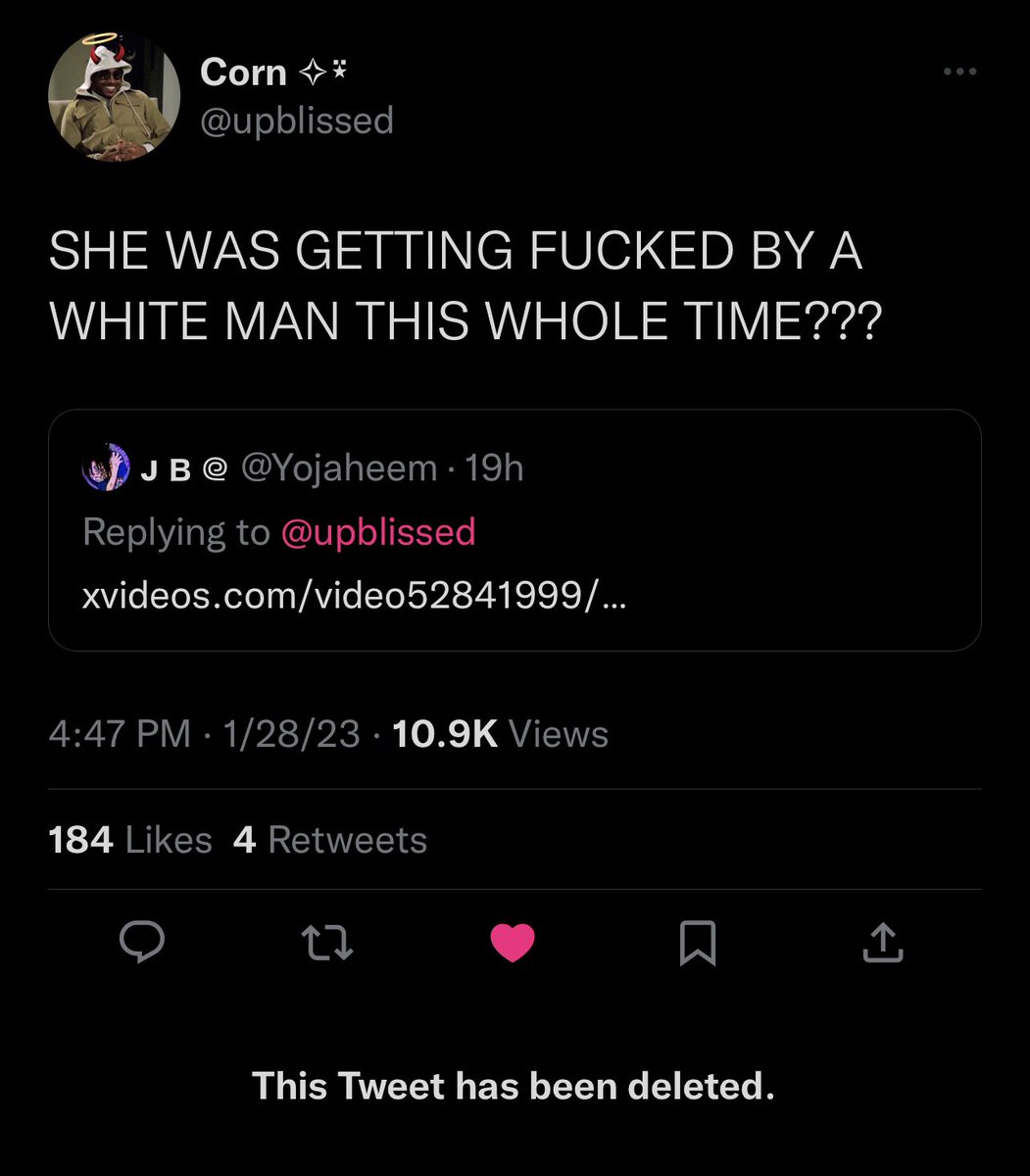Here’s a cleaned-up and detailed caption for the described image:

---

This image is a screenshot from Twitter featuring a black interface. In the top left corner, there is a profile picture of an individual wearing a hat, adorned with whimsical ears and a halo, labeled with the name "Korn" and various small icons next to it. Directly below, in a large white font, a provocative statement reads: "She was getting f'd by a white man this whole time???".

In response to this tweet, there is a secondary icon labeled "jb." Alongside this is the handle "@yojaheem," marked with a timestamp "19h" and indicating a reply to "@up_blist". An accompanying URL is provided: "xvideos.com/video52841999/...". 

Further details below this response include the timestamp "4:47 PM, 1/28/23" and a view count of "10.9k views." Interaction metrics display "184 likes" and "4 retweets." Underneath, there are icons for sharing, tagging, liking, and commenting, totaling five in number.

At the bottom of the screenshot, a notation indicates: "This tweet has been deleted."

---

This caption captures the key elements and context of the original image while providing a clear, descriptive overview.